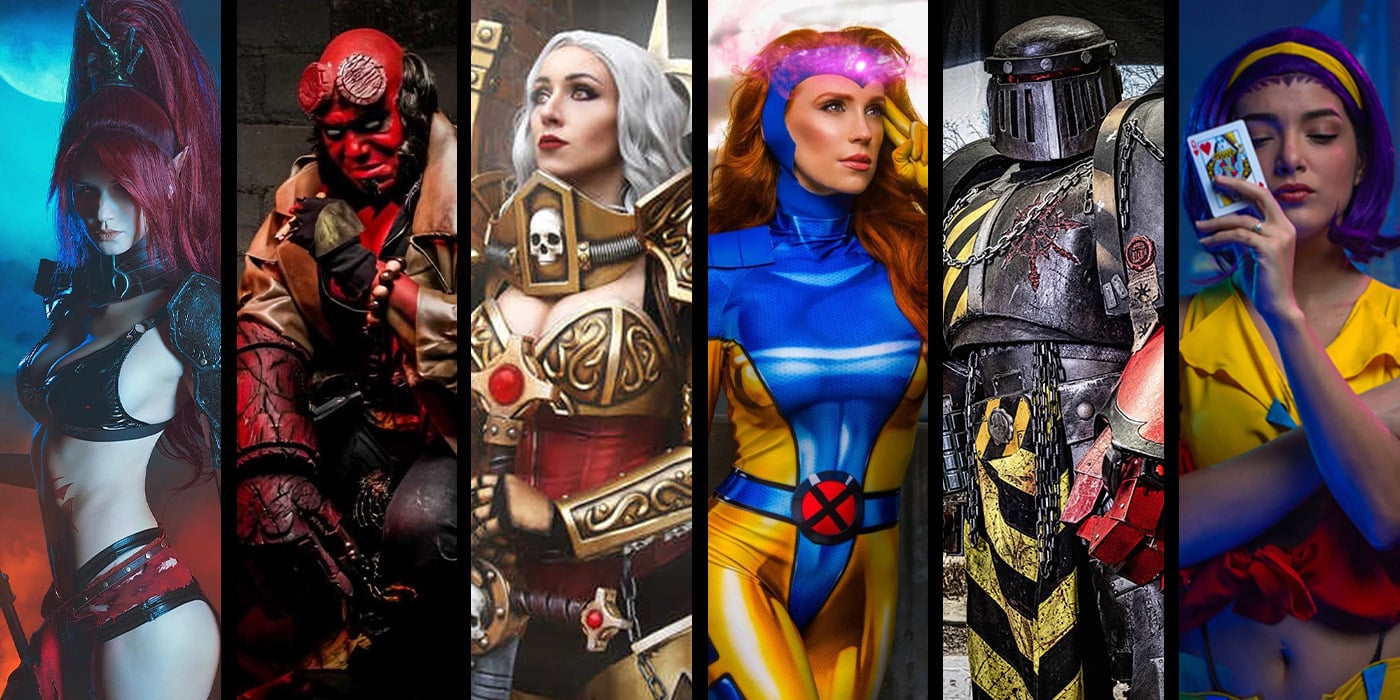The image is a horizontally oriented composite divided into six vertical sections, each depicting a distinct character from a fantasy realm. From left to right:

1. **Tall Female Warrior**: A striking woman with vibrant red hair tied in a high ponytail, dressed in a revealing black PVC bikini top and high-waisted red panties accentuated with black leather straps. She displays her pale abdomen and wears a collar around her neck. The background features a mystical blue moon or planet amidst a red and blue sky.

2. **Red-Skinned Male**: A crouching male figure with red skin, white eyes, and goggles perched above his eyes. He sports a thick golden jacket, black leather trousers, and a large beaded necklace around his wrist. His thick black beard and the mechanical red glove highlight his rugged appearance.

3. **White-Haired Female Warrior**: This female character boasts wavy white hair, elaborate gold armor on her arms, and a busty golden bra top with a red corset. She wields a sword adorned with a red dot and skull at the hilt, wears a gold skull necklace, and gazes into the distance with prominently made-up eyes and red lipstick.

4. **Heroic Female in Bodysuit**: She stands in a blue and gold catsuit with a prominent turquoise cross pattern on the chest extending to her right ear. Her pink hair, a glowing purple gem on her forehead, and yellow gloves add to her striking presence as she points her fingers to her temple, also looking into the distance.

5. **Armored Knight**: Encased in full metal armor, this faceless character features black and yellow striped fabric and numerous chains draped from the waist and neck. A red mechanical arm and hand peek out, adding to the imposing and enigmatic appearance.

6. **Mystical Female**: The final character is a serene woman with a bob haircut in purple, adorned with a golden headband. She holds a Queen of Hearts card close to her face, eyes closed, and wears a yellow top with a ruffled red bottom that exposes her stomach and belly button.

This detailed composition captures the essence and diversity of characters from a fantastical universe, each bringing their unique attributes and mystique to the ensemble.